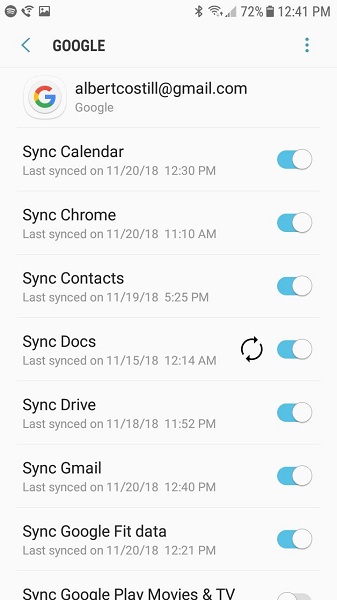The image is a detailed screenshot of a person's cell phone, displaying a portion of their Google account settings. At the top of the screen, typical cell phone status icons are visible, including Bluetooth, Wi-Fi, cellular data, and battery level, which shows 72% remaining. The time displayed is 12:41 p.m.

Below the status bar, the screen prominently features Google settings. At the top left, there is a Google 'G' logo, with the email address albertcostille@gmail.com displayed next to it. The heading below reads "Google." This section pertains to the synchronization settings between the user's computer and cell phone.

The sync settings are listed as follows:
1. **Sync Calendar** - Last synced on 11/30/18 at 12:30 p.m.
2. **Sync Chrome** - Last synced on 11/20/18 at 11:10 a.m.
3. **Sync Contacts** - Last synced on 11/19/18 at 5:25 p.m.
4. **Sync Docs** - Last synced on 11/15/18 at 12:14 a.m. (Indicated by two arrows forming a circle, showing it is still syncing.)
5. **Sync Drive** - Last synced on 11/18/18 at 11:52 p.m.
6. **Sync Gmail** - Last synced on 11/20/18 at 12:40 p.m.
7. **Sync Google Fit data** - Last synced on 11/20/18 at 12:21 p.m.

All the aforementioned sync options are toggled on, indicated by blue ovals with a white circle on the right-hand side. The final option:
8. **Sync Google Play Movies and TV**

This option is toggled off, marked by a gray oval with a white circle on the left.

There is no additional text or information provided on the screen.